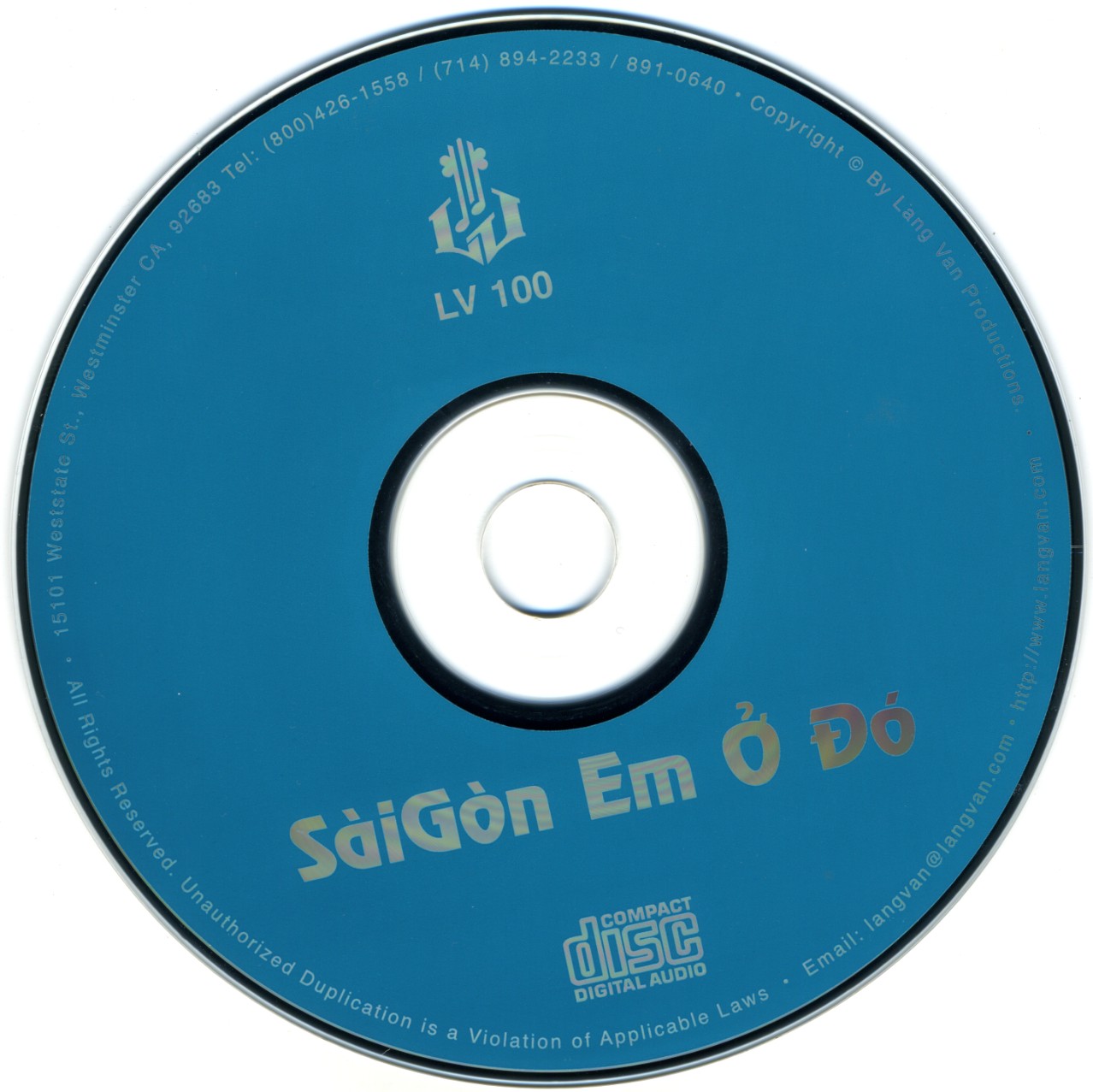This image captures a vintage compact disc (CD), predominantly blue in color. The CD features the text "Saigon M. O'Do" at the bottom, which might refer to either the band or the album title. Above this text, there is a symbol accompanied by the designation "LV-100". The central region of the CD is white, contrasting with the blue expanse of the disc. The disc has the characteristic central hole designed to fit onto a CD player spindle, allowing it to spin during playback.